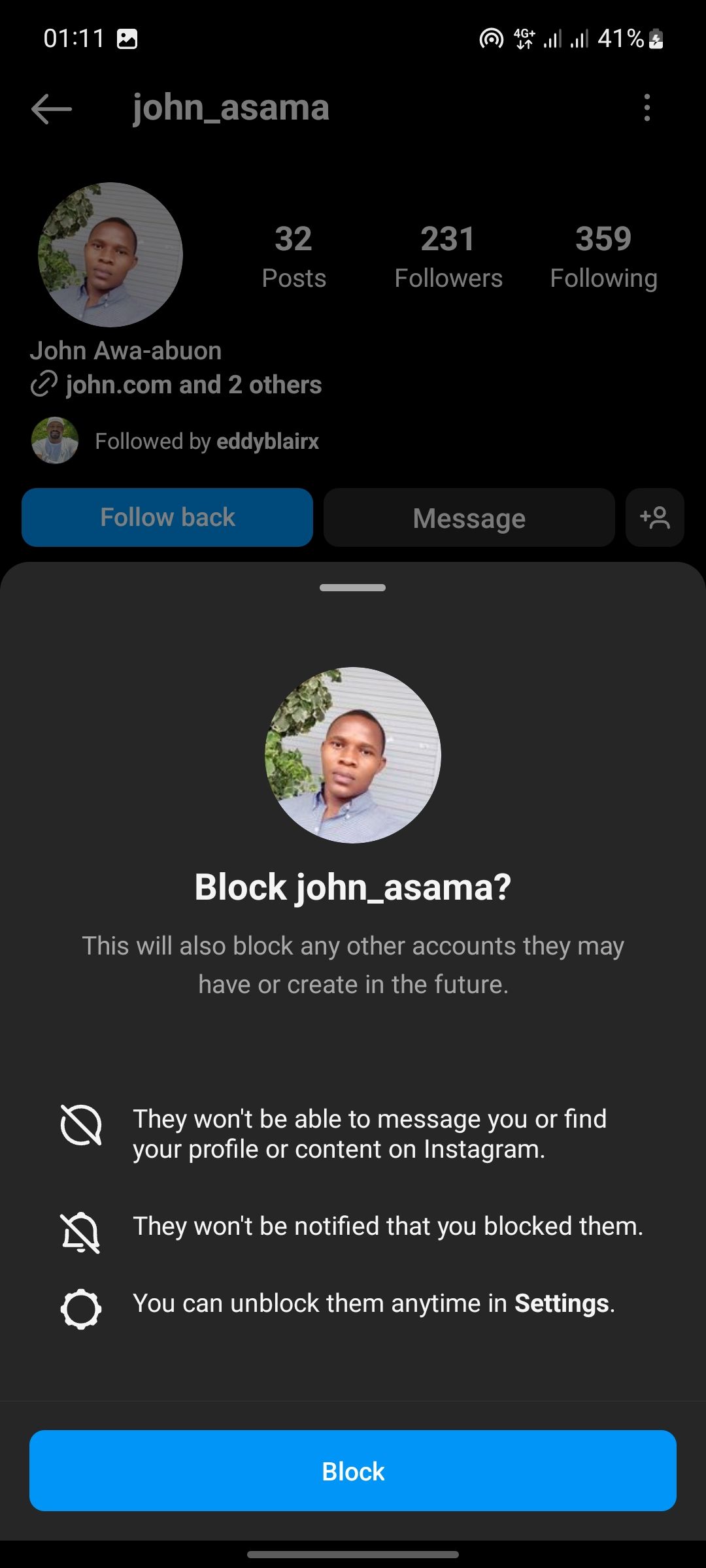The image is a screenshot captured in portrait mode. At the top-left corner, the time is displayed as 1:11, while the top-right corner shows the battery level at 41%. The next row features the name "John Asama." Below it, there's an avatar of John—a dark-skinned man wearing a blue button-up shirt, positioned next to green leaves within a circular frame. His profile details indicate that he has made 32 posts and has 231 followers, while he is following 359 accounts. 

The account name is displayed as "John Awa Abun," followed by a link to "John.com" and two other unspecified links. The profile is also followed by Eddie Blair X, with an option to "Follow Back" in blue, suggesting a pending follow request.

Further down, there's an option to message John Asama and another option to "Block" him. A detailed explanation follows, stating that blocking John Asama will block any future accounts he might create and prevent him from messaging, finding, or viewing your profile and content on Instagram. It also reassures that John won't be notified about the block and that the user can unblock him anytime in settings.

At the bottom of the screen is a prominent blue button labeled "Block," implying the user has accessed Instagram's block feature, possibly viewing this screen due to concerns over the authenticity of John's account or a lack of interest in engaging with him.